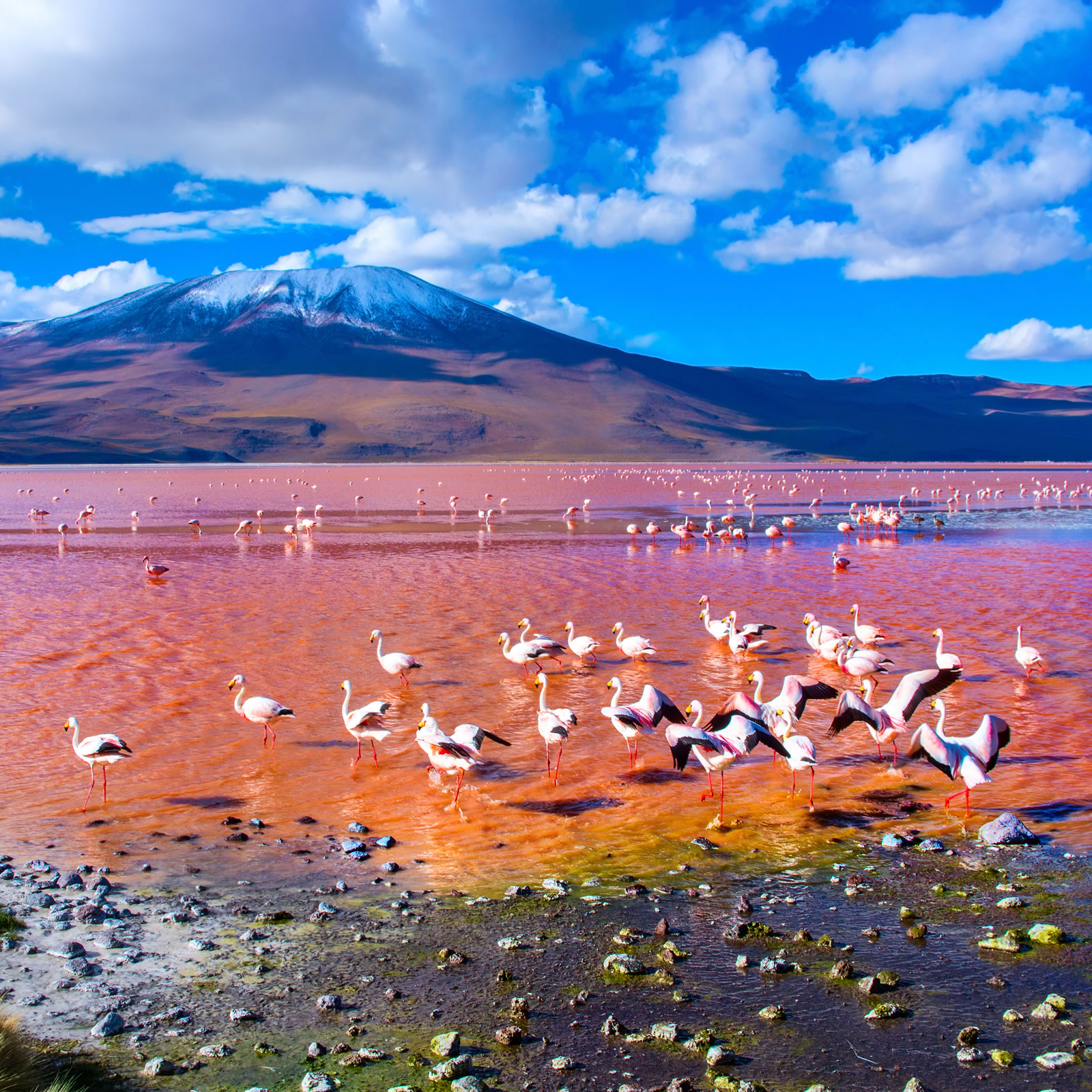In the foreground of the photograph, a multitude of tall white birds, possibly flamingos with black-tipped wings, are congregated in the shallow, reddish-hued waters of a lakeside beach. Their long, slender legs navigate through the wet, rocky terrain scattered with shells and moss. As the eye moves beyond the birds, the water deepens and takes on a richer red tone, blending into a tranquil scene. In the background, a stark blue sky with occasional clouds stretches above distant, snow-capped mountains, creating a picturesque and serene atmosphere. This landscape captures a peaceful moment with hundreds of birds enjoying their day in the uniquely colored water against a backdrop of natural beauty.